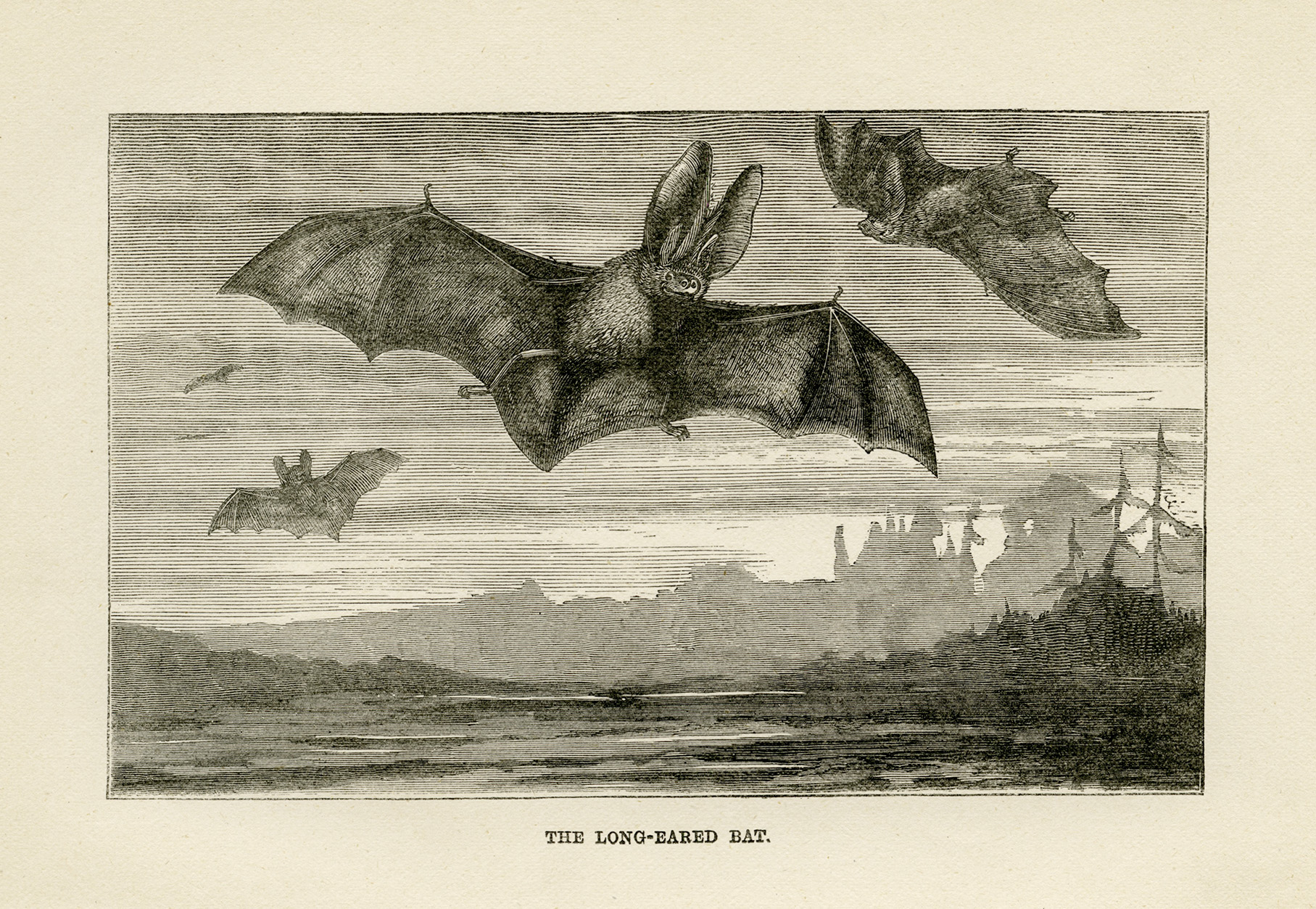This is a black and white framed pencil drawing titled "The Long-Eared Bat." At the center of the artwork, a large bat with distinctly long ears is depicted with its wings fully outstretched, showcasing intricate details. To the right of this primary bat, another bat is shown in flight from a top view, and to the left, a smaller bat is depicted flying with its wings extended. In the background, there are less detailed, tiny bats scattered across the night sky. The lower section of the drawing features a landscape with sparse details suggesting trees, mountains, and possibly housing units. Additionally, there is text at the bottom of the image, in all capital letters, that reads "THE LONG-EARED BAT."